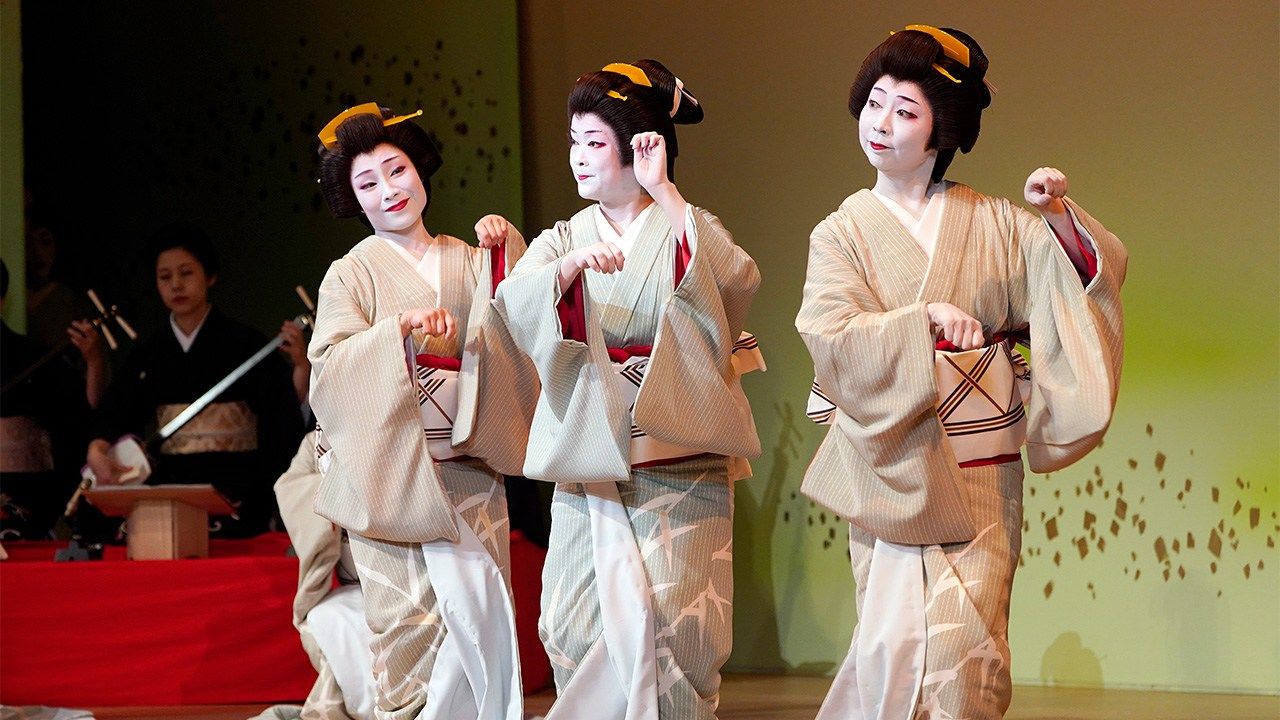This photograph captures a vividly lit performance featuring three Japanese geishas. The geishas, adorned in traditional beige robes with white undergarments and accented with red fabrics, have their faces painted white, with bright red lips and eye makeup that highlights their eyes. Their black hair is styled up, held in place with distinctive orange accessories. The two geishas on the right display a facial expression with puffed cheeks and tight lips, while the one on the left smiles softly, gazing at her companions. All three women have their wrists elegantly raised to their right side, engaging in a synchronized dance. In the dimly lit background on the left, a person, potentially another performer, holds a musical instrument, likely contributing to the musical ambiance of the performance. The backdrop features a mix of gray, brown, and yellow hues, accentuating the scene's traditional yet theatrical atmosphere.